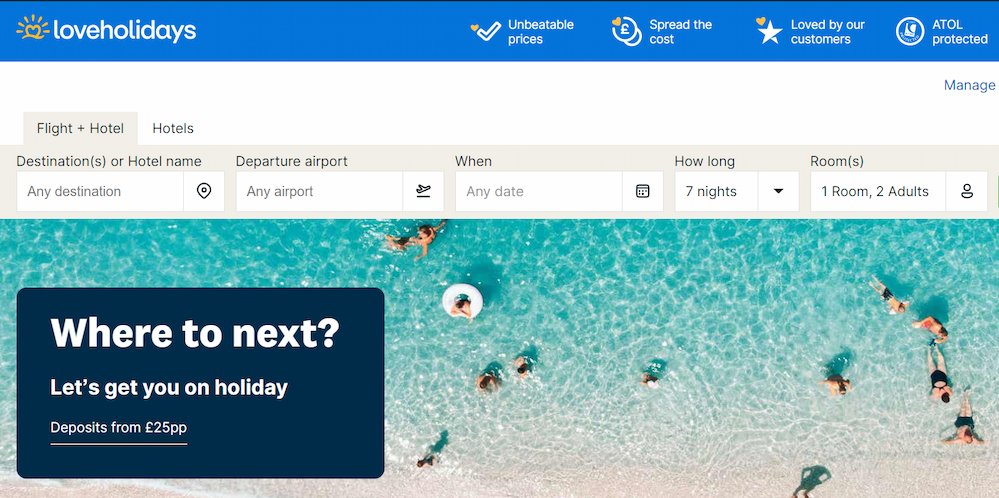Here is a refined and detailed caption for the image:

---

The image captures the Love Holidays website's header and search interface. The brand's name "Love Holidays" is prominently displayed on the upper left-hand side in lowercase white font. Accompanying the text is a logo featuring a heart with a wavy line at the bottom and a curving line at the top, giving the impression of rays emanating from the heart. This logo and text are set against a blue bar that spans the width of the screen.

Within this blue bar, several key selling points are highlighted: "Unbeatable Prices," "Spread the Cost," "Loved by Our Customers," and "ATOL Protected." Just below, there are two tabs to choose the type of booking: "Flight + Hotel" and "Hotel," with the "Flight + Hotel" tab currently selected.

Directly beneath these tabs is a series of input fields for planning a trip. The first field is for entering destination names or hotel names ("Any Destination" is the placeholder text). Next, there is a field for selecting the departure airport, labeled "Departure Airport" with a placeholder of "Any Airport." This is followed by the "When" box, allowing users to input travel dates, with "Any Day" as a placeholder. The next field is labeled "How Long," with "7 Nights" pre-filled as the default option. Finally, there is a "Room" section specifying one room and two adults as the current selection.

---